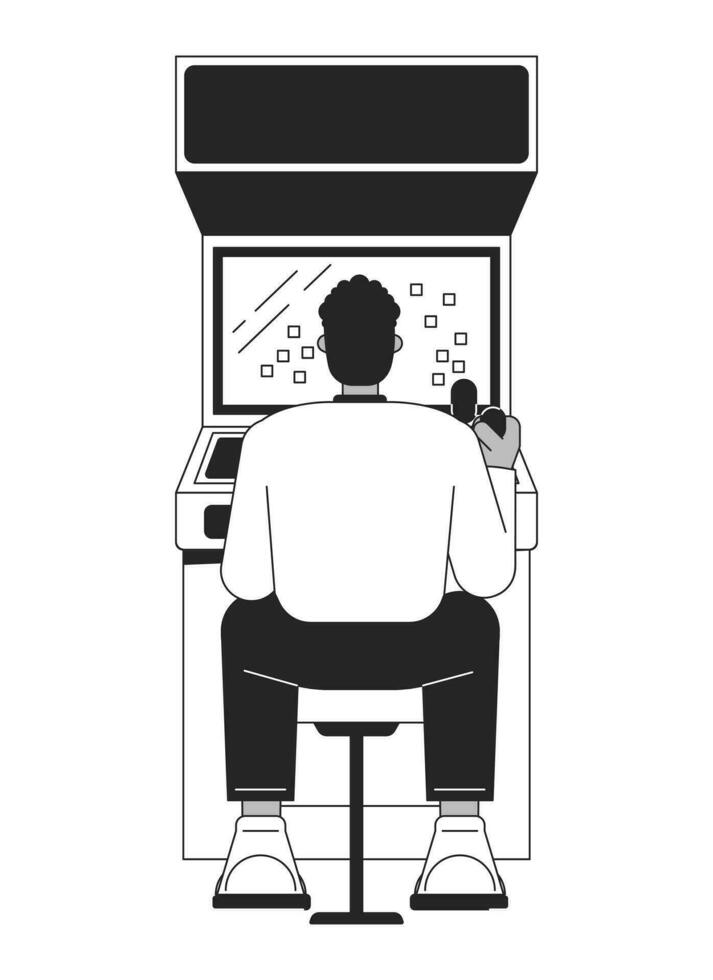This black-and-white line drawing features a man with a large frame sitting on a white stool in front of an arcade machine. His back is turned to the viewer as he intently gazes at the arcade screen. With curly black hair and ears visible on either side of his head, he is dressed in a long-sleeved white shirt with a black collar, black pants, and white shoes with black soles. The man holds a black joystick in his right hand, while his left hand is not visible. The arcade machine is depicted with a solid black rectangle at the top where the game logo would be, and the screen shows several small squares with diagonal motion lines, suggesting in-game action. The overall style of the image emphasizes the simplicity and nostalgic ambiance of classic arcade gaming.